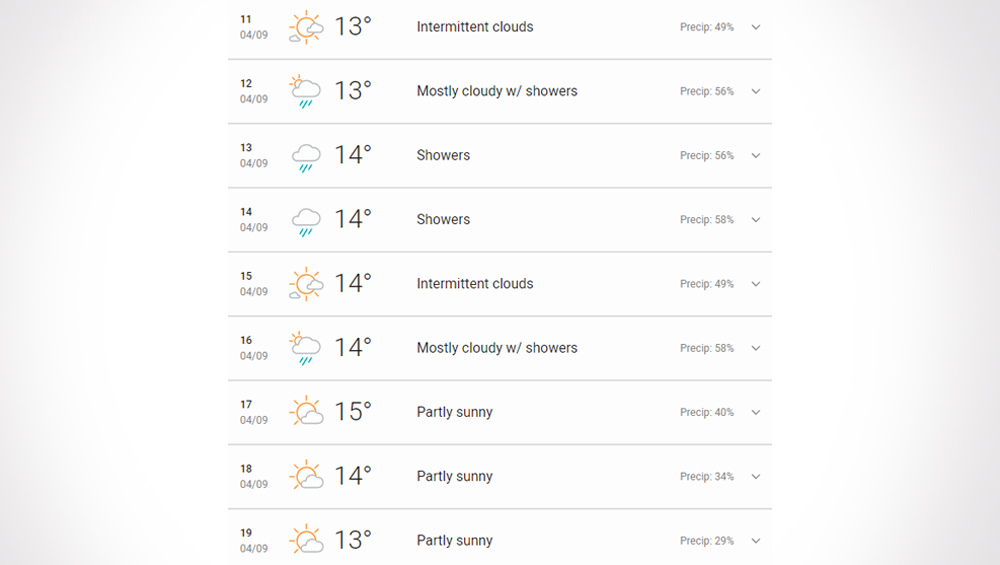This detailed screenshot captures an hourly weather forecast for an unspecified location on April 9th, without indicating the year. The temperatures are likely given in degrees Celsius. The forecast spans from 1:00 PM to 7:00 PM, with conditions fluctuating between intermittent clouds, showers, and partly sunny skies. 

1:00 PM - Temperature: 13°C, Intermittent clouds, 49% chance of precipitation.
2:00 PM - Temperature: 13°C, Mostly cloudy with showers, 56% chance of precipitation.
3:00 PM - Temperature: 14°C, Showers, 56% chance of precipitation.
4:00 PM - Temperature: 14°C, Intermittent clouds, 49% chance of precipitation.
5:00 PM - Temperature: 14°C, Mostly cloudy with showers, 58% chance of precipitation.
6:00 PM - Temperature: 15°C, Partly sunny, 40% chance of precipitation.
7:00 PM - Temperature: 14°C, Partly sunny, 34% chance of precipitation.
8:00 PM - Temperature: 13°C, Partly sunny, slight chance of showers. 

The relatively low temperatures suggest that the temperature readings are likely in Celsius. Despite the cooler weather, there remains a varied chance of precipitation throughout the timeframe.